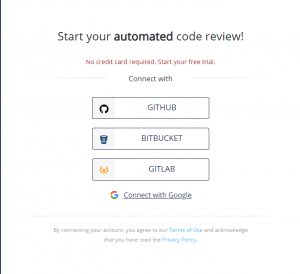The screen features a white background with a centralized focus where a concise prompt and a message are displayed. At the top, in bold black font, the text reads: "Start Your Automated Code Review!" with "Automated" emphasized in bold. Directly below, in red font, it states: "No credit card required. Start your free trial."

Beneath this message, users are presented with three options to connect their accounts, each placed in a distinct bar with corresponding icons on the left:
1. GitHub: Represented by a black circle containing a white plug icon.
2. Bitbucket: Illustrated with a blue bucket icon.
3. GitLab: Depicted with a yellow fox head icon.

An additional option to connect with Google is located below these three choices. It features a multicolored "G" logo followed by the text "Connect with Google."

At the bottom of the screen, a final message reads: "By connecting your account, you agree to the Terms of Use and acknowledge that you have read the Privacy Policy." The phrases "Terms of Use" and "Privacy Policy" are highlighted in blue font for emphasis.

The screen also includes subtle design elements: two faint gray lines frame the "Connect with" options, and another faint gray line appears above the final message at the bottom of the screen.